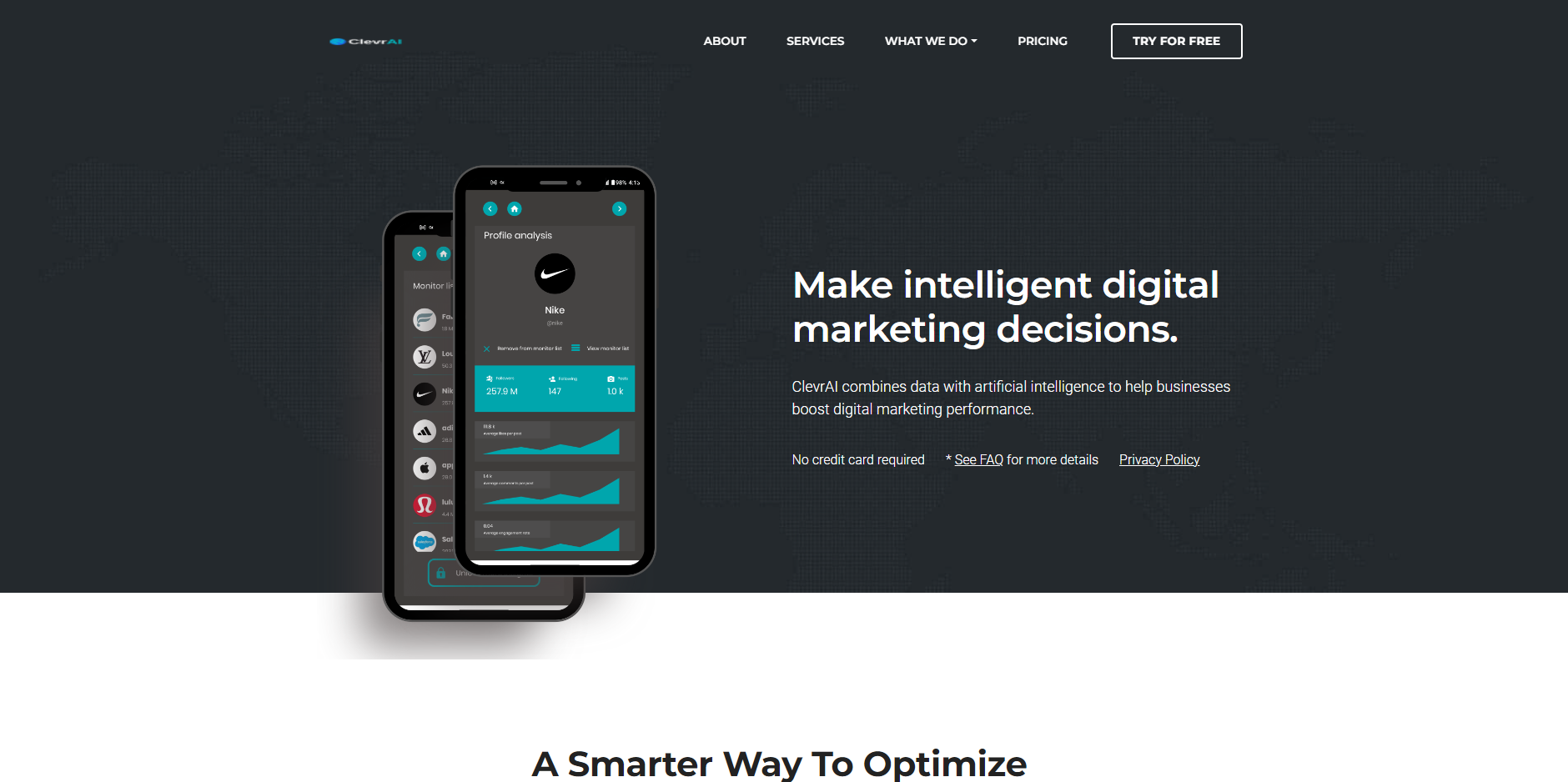This screenshot captures a web page with a predominantly dark gray background, occupying approximately three-quarters of the screen. In the upper left corner, the company name "Clever AI" is displayed, though it is somewhat hard to see. "Clever" is written in white letters, while "AI" is adjacent in blue letters, accompanied by a small blue oval shape to the left of the name.

Towards the center of the page is the main navigation menu, presented in white font. The menu includes options such as "About," "Services," and "What We Do," with an inverted triangle indicating a drop-down menu. Additional options include "Pricing" and "Try for Free," the latter being enclosed in a white-lined rectangle.

Central to the page is an image showcasing two smartphones stacked atop one another, displaying the product’s dashboard. Both screens have very dark gray backgrounds featuring graphs and charts in a turquoise-blue hue.

On the right of the smartphones, bold white text states, "Make intelligent digital marketing decisions." Below this, regular, non-bold text reads, "Clever AI combines data with artificial intelligence to help businesses boost digital marketing performance." It also mentions, "No credit card required," and directs users to "See FAQ for more details," with "FAQ" being an underlined, clickable link. Similarly, "privacy policy" is hyperlinked and underlined.

At the bottom of the page, the background turns white. Centered in black font are the words, "A smarter way to optimize."